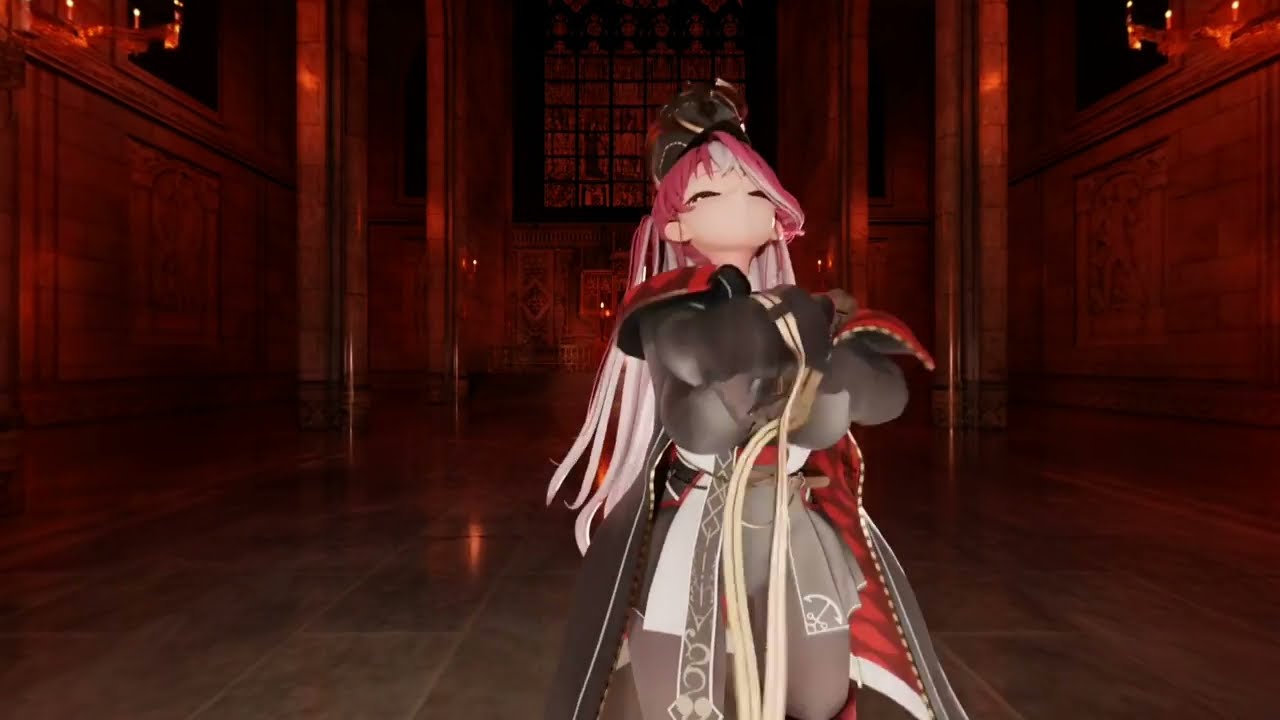The image depicts a digitally-rendered character, resembling an anime-style figure, centered within a dimly-lit, expansive hallway that gives the impression of a large building, possibly a palace. The character, a young girl with distinctive pink hair that transitions to white, fair peach skin, and a contemplative expression, stands out prominently. She is adorned in a red and black robe over gray pants, cinched at the waist with a brown belt, suggesting a possible warrior or princess-like persona.

Her surroundings include a stone floor that stretches below her, adorned with what appears to be rugs or tapestries adding to the Oriental or Asian aesthetic of the scene. Twin light fixtures, possibly candles, are situated on either side of the image near the upper corners, casting a reddish glow that envelops the entire backdrop in a dark, golden-orange hue. Behind her, tall walls rise upward, suggesting vast ceilings, and in the distance, there might be a large stained glass window, adding a majestic feel to the setting. The scene combines elements of both a lifelike photograph and a computer-generated imagery, creating a surreal, almost lifelike appearance.